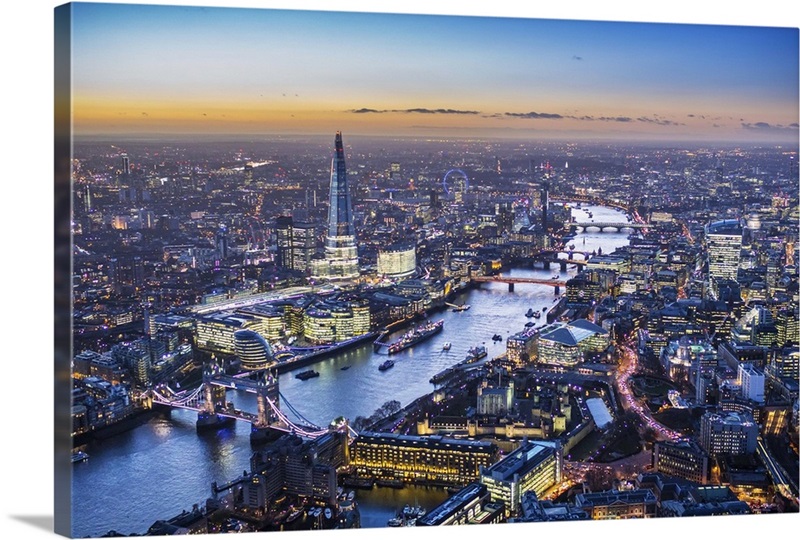This detailed image is a color photograph printed on a 3D canvas that wraps around a boxy frame, depicting a panoramic aerial view of a riverfront city, most likely London, during dusk or twilight. The River Thames runs prominently through the center of the city, with at least five bridges, including one that resembles London Bridge, festooned with lights on its cables and pillars. The scene is brilliantly illuminated with city lights, streaming from buildings and street traffic. The skyline is a mix of tall skyscrapers and large buildings, including iconic structures such as the London Eye in the background and the Shard, a highly distinctive, tall pyramid-shaped building. The photograph captures subtle transitions in the sky from light blue to a yellowy-orange, indicative of a setting sun, with some scattered darker clouds. The river itself hosts a variety of vessels, from large ships to small boats. In the foreground, a notably curved building is well lit, alongside numerous other buildings and highways alive with the lights and movement of city life. The background stretches out into a blurred expanse of blue-gray urban landscape, peppered with the glow of distant city lights.